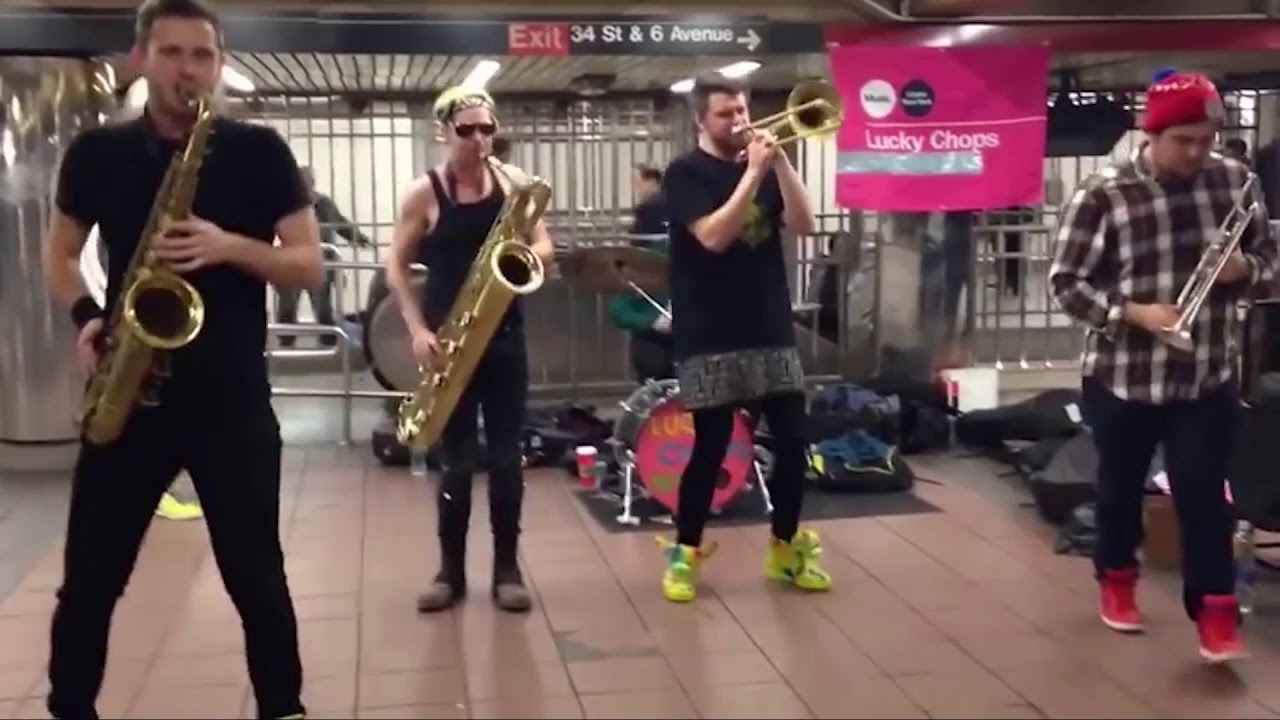In this detailed color photograph, we see a four-piece band of street musicians performing in a subway station. The band, comprised of four men aged in their late 20s to early 30s, are all standing with their instruments ready. On the left, a man wearing a black t-shirt, black pants, and a black wristband is playing a saxophone. To his right, a second man, donning a black sleeveless t-shirt, dark shades, and black trousers, is playing a larger bass saxophone. Next, a man with a black t-shirt and green shoes is playing a trombone. Finally, on the far right, a man is playing a silver trumpet, dressed in a brown shirt, red beanie, and matching red shoes. 

Behind the musicians, a drum set is partially visible alongside some bars and a metal grate extending from the ceiling to the ground. A pink banner with white text that reads "Lucky Chops" hangs prominently in the upper right corner. The beige tile floor and evident details place the performance in a subway station, captured in a photographic representational realism style. The band members, despite the underground setting, convey a vibrant and composed presence, making the image a compelling snapshot of urban street performance.